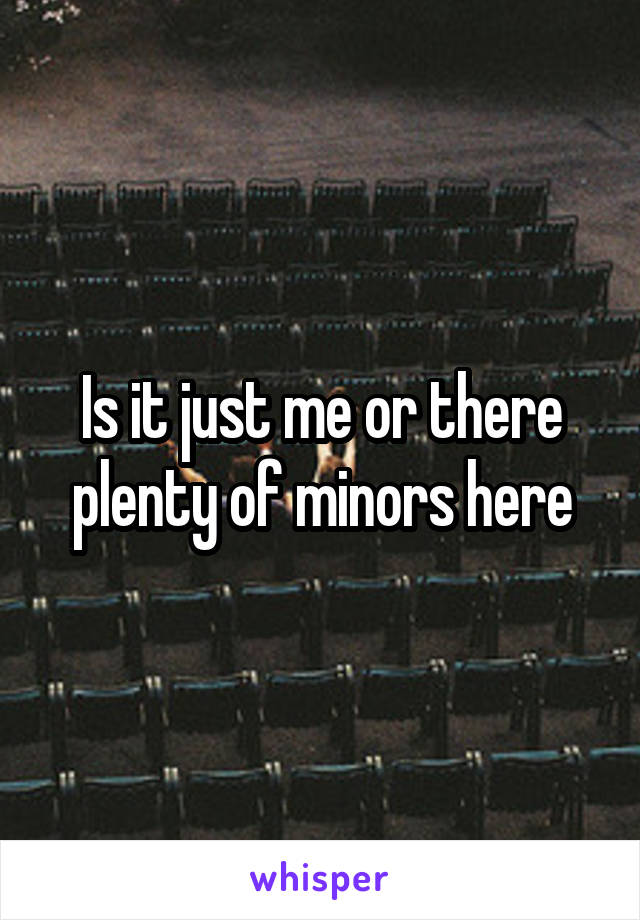This image depicts an aerial view inside a concert hall or theater featuring numerous rows of black chairs, suggesting it could be a large public venue such as a stadium or concert hall. The seating area is punctuated by a couple of individuals who appear to have their feet up on chairs in front of them, though their details are obscured by an overlay of text. The setting shows a stark contrast between a tan and black backdrop. The concrete flooring is visible in front of the seating arrangement. Across the center of the image, a caption in skinny white font with a black outline reads, "Is it just me or are there plenty of minors here?" Below this, there is a small white banner with the word "whisper" written in lowercase purple letters. The overall scene is reminiscent of a meme or social media post, characterized by its specific use of text and imagery to convey a subtle or humorous message.